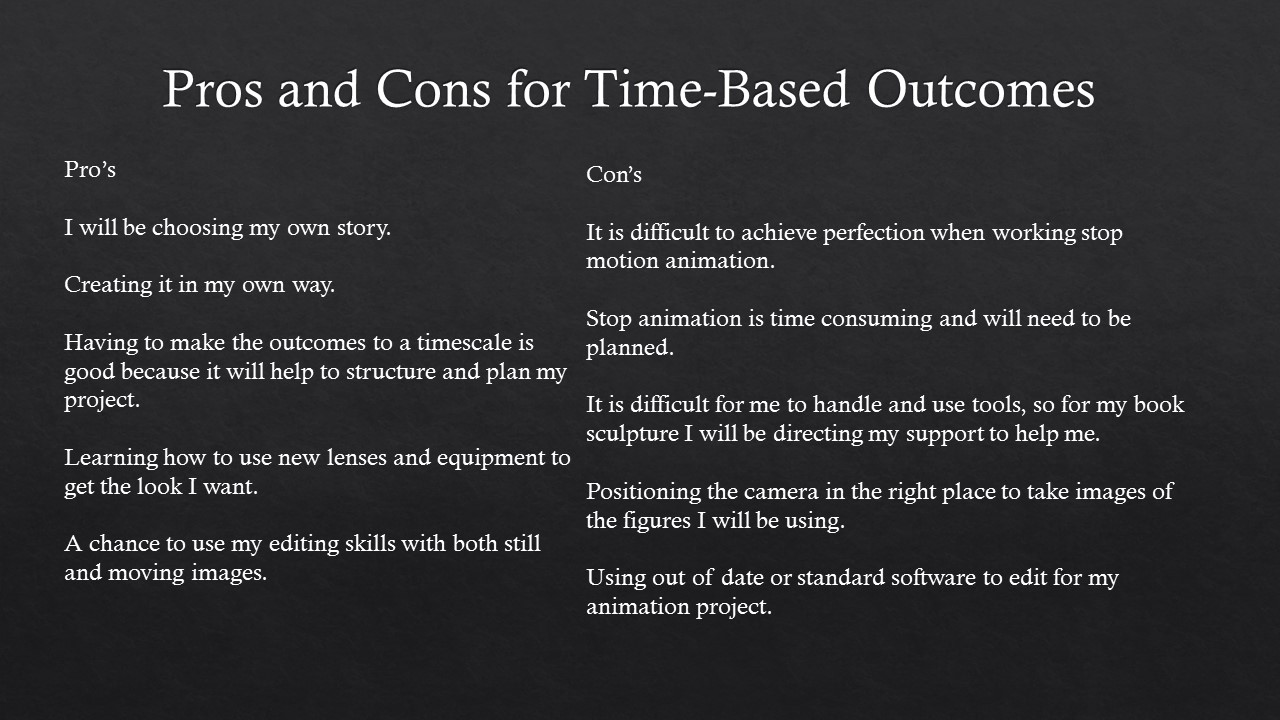The image is a black and white graphic with a black background and white text, titled "Pros and Cons for Time-Based Outcomes." The title is prominently displayed at the top in bold letters. Below the title, the content is split into two columns: "Pros" on the left and "Cons" on the right. 

Under "Pros," the list includes:
- "I will be choosing my own story, creating it in my own way."
- "Having to make outcomes to a time scale is good because it will help to structure and plan my project."
- "Learning how to use new lenses and equipment to get the look I want."
- "A chance to use my editing skills with both still and moving images."

Under "Cons," the list mentions:
- "It is difficult to achieve perfection when working with stop-motion animation."
- "Stop-motion animation is time-consuming and will need to be planned."
- "It is difficult for me to handle unused tools, so for my book sculpture I will be directing my support to help me."
- "Positioning the camera in the right place to take images of the figures I will be using."
- "Using out-of-date or standard software to edit for my animation project."

The overall design resembles a PowerPoint slide, pamphlet, or wall hanging, devoid of any objects and featuring only text presented in a clear and structured format.